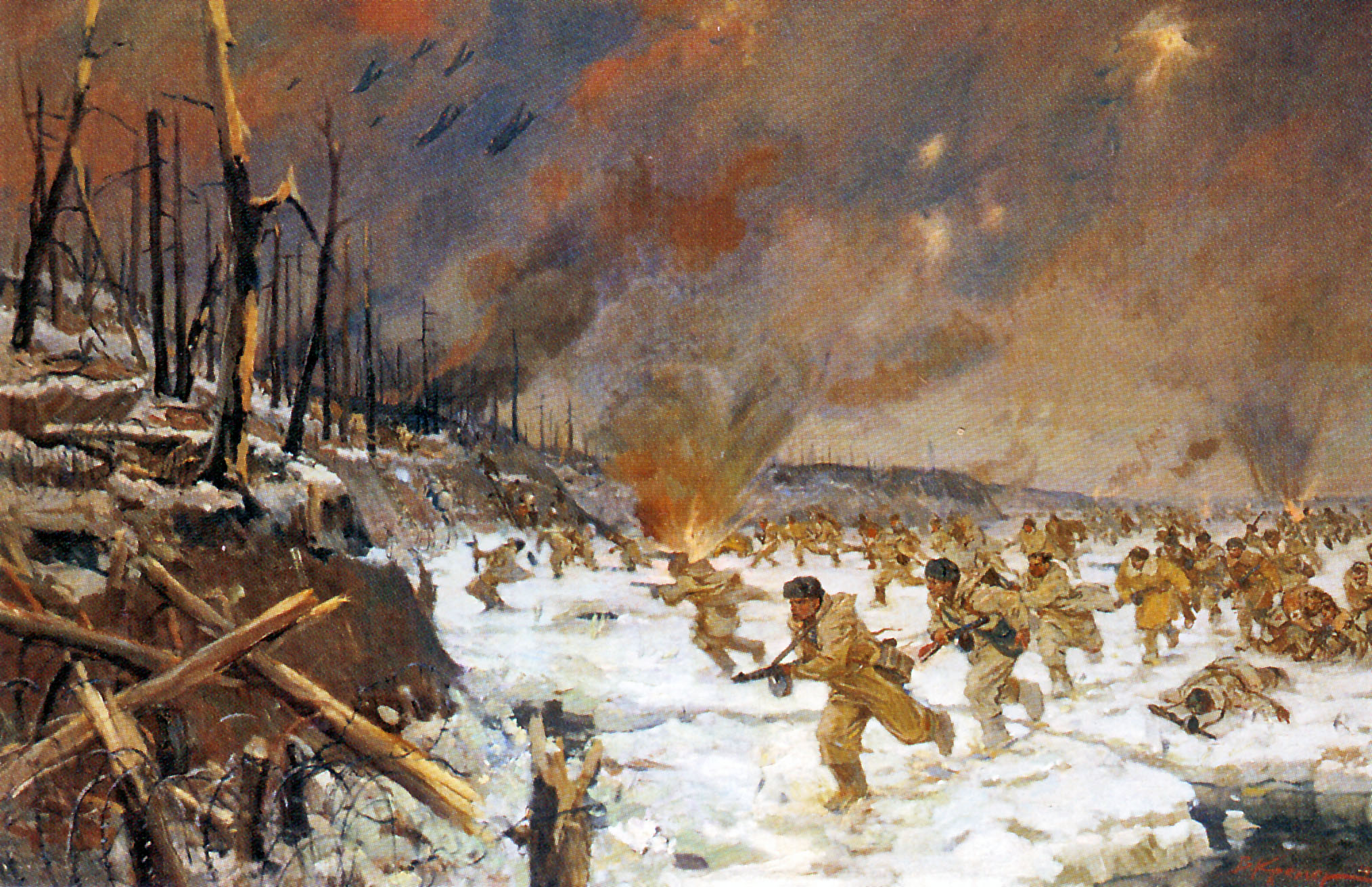The image portrays a harrowing scene of a World War II battle in a snowy, wintry setting. The ground is covered with snow, and the sky is a turbulent mix of dark, smoky gray and blue, punctuated by fiery explosions and the glow of orange flames. Soldiers in heavy-duty warm coats, pants, and boots are seen rushing from right to left, carrying rifles and advancing toward a leafless, barren forest. The trees, which are thin and appear damaged, likely burnt out or bombed, stand as stark sentinels in the background. Barbed wire is strewn across the snow-covered ground, and planes loom ominously in the smoky sky above. Among the chaotic scene, some soldiers are depicted falling as if they've been shot, adding to the intense atmosphere of the battle. The painting includes a signature in the bottom right-hand corner, though it's slightly blurry and hard to decipher. The overall color palette involves a dirty white snow, brown tones, shades of blue in the sky, and the fiery oranges of the flames, creating a vivid and dynamic portrayal of wartime hardship.